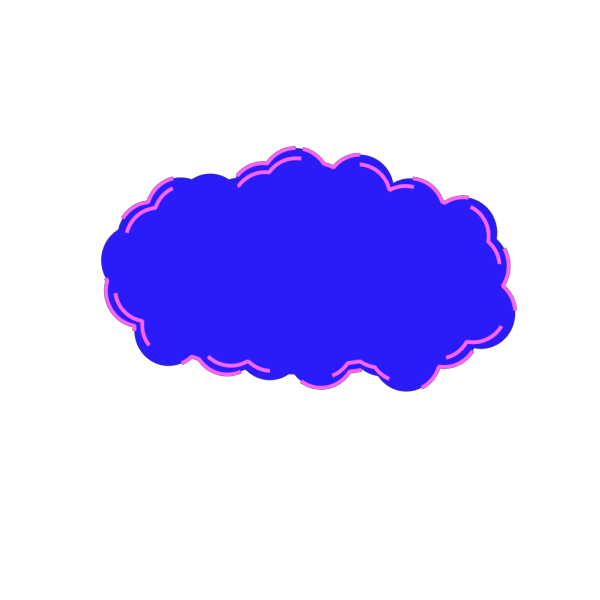The image depicts a simple digital illustration of a vibrant blue cloud set against a completely white background. The cloud is horizontally oblong, with a very curvy, lumpy outline. Its edges are emphasized by irregularly placed, vibrant light purple or pink neon lines, both along some of the outer curves and slightly within the edges, adding texture and highlighting the cloud's shape. Though these neon lines don't fully enclose the cloud, they accentuate its distinctive, rounded form. Overall, the image is plain yet vivid, focusing solely on the intricately detailed blue cloud.